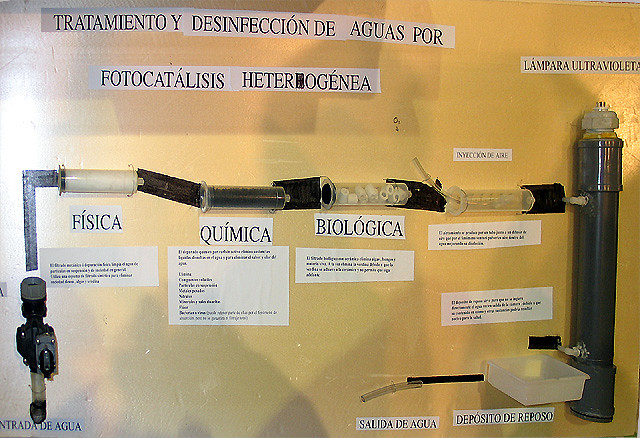The image captures a horizontally aligned rectangular scene featuring a contraption affixed to a yellow wall. This setup consists of several interconnected tubes, some clear and others dark-colored, arranged both vertically and horizontally. Central to the display is a prominent tall gray cylinder on the right side, leading into various other containers and cylinders, which include dark and clear components filled with cut-up shapes resembling pieces of PVC pipe. Below this array is a tray, possibly part of a control valve assembly.

Above the apparatus are several large rectangular strips of paper with Spanish text printed on them. The top title reads, "Tratamiento y Desinfección de Aguas por Photocatalysis Heterogenea," which indicates a focus on water treatment and disinfection through heterogeneous photocatalysis. Further down, some individual labels next to the gadget are marked "Física," "Química," and "Biológica," suggesting different scientific categories related to the contraption’s function. Additionally, larger sheets with smaller black text provide further descriptions, though they are not legible in the image. The entire assembly looks intricate, indicative of a specific technical or scientific process.